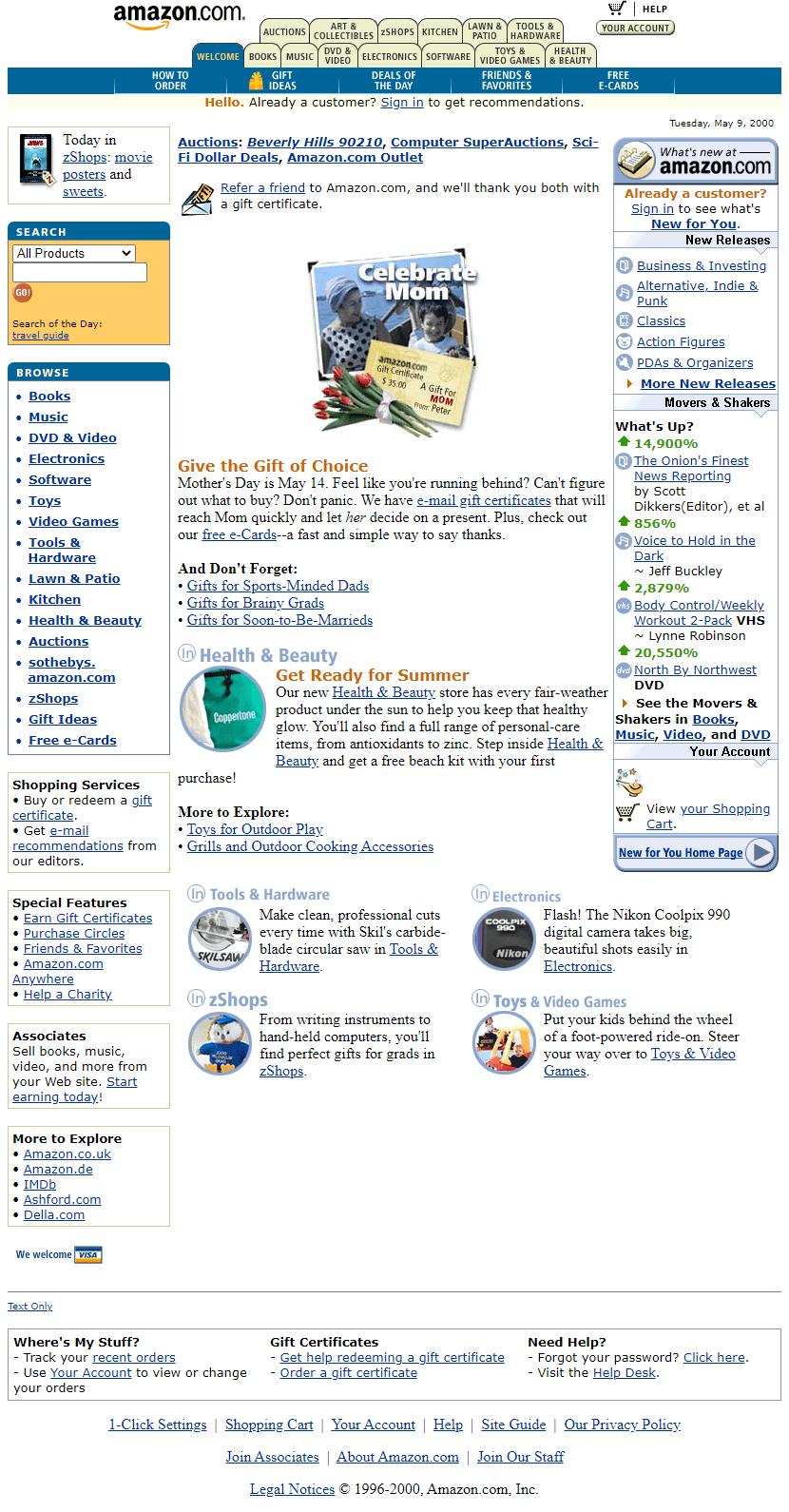The image is a historical screenshot from Amazon.com, dated Tuesday, May 9, 2000, making it over 23 years old. The webpage reflects the primitive design standards of that time, characterized by plain and somewhat uninspiring text without any video elements. Sparse images punctuate the text-heavy layout, which can appear overwhelming due to the small font size and dense information.

At the top of the page, a promotional banner highlights the upcoming Mother's Day on May 14, urging users to "Celebrate Mom" and "Give the Gift of Choice." The page structure includes various navigational links on both sides: a browsing section and search bar on the left, and sections for new releases, movers and shakers, and user account management on the right.

Overall, the design is cluttered and lacks the sophisticated visuals and user-friendly navigation typical of modern websites, reflecting the nascent stage of e-commerce design at the turn of the millennium.